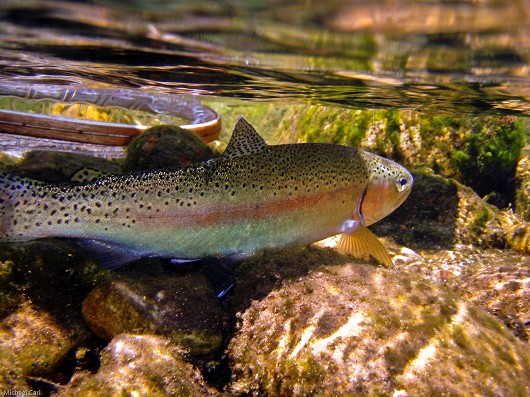In this captivating photograph, we observe a fish with a distinctive pale yellow body adorned with black spots on its upper half and a red line accentuating its greenish bottom. The fish appears near the surface of a crystal-clear, shallow water area, possibly close to the bank of a pond, river, or lake. Below the fish, we see an array of rocks that almost touch its belly, illustrating the shallowness of the water. The water itself is remarkably transparent, revealing everything underneath with striking clarity, including patches of green algae and various aquatic plants. Nearby, there is a slithering entity, possibly a snake or an eel, weaving through the water. To the left of the fish, a circular structure is visible, which might be a net or part of photography equipment aimed at capturing this serene aquatic scene.